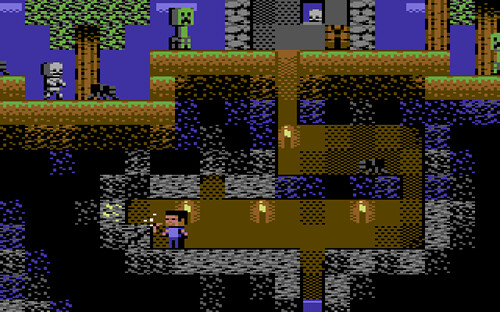The image is a horizontally-oriented screenshot from an early 1990s video game, featuring retro, pixelated graphics reminiscent of classics from the late 1980s. The main character is navigating a labyrinthine underground environment, moving leftward through a network of tunnels. Above the tunnels, menacing undead creatures loom, including a green face with a frown, a creature resembling a spider, and several grey, skeletal figures. The graphics are rudimentary yet charming, reflecting the technological limitations of the era. The color palette primarily consists of blue, black, and brown, with splashes of green to highlight the living entities. The gameplay appears to involve guiding the main character through the tunnels, skillfully avoiding or confronting foes along the way.